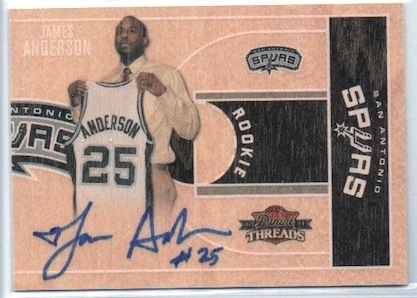This detailed description amalgamates the shared and repeated details with emphasis on clarity:

This is a rookie basketball card for James Anderson of the San Antonio Spurs, capturing the moment he received his first jersey, number 25. The card features Anderson facing the viewer, wearing a button-down shirt and tie along with light brown pants. He holds up his black and white Spurs jersey, which prominently displays "Anderson 25." The card includes Anderson's autograph in blue ink positioned at the bottom left. Above his head and slightly to the left, his name, "James Anderson," is written, with additional text indicating his rookie status and displaying the Spurs' logo in multiple locations on the card. The background largely employs pink with black and white elements from the Spurs' colors, and orange tones are seen near a basketball image on the card. The card is produced by P-A-N-I-R-I Threads, indicated underneath the photograph, and the design hints it might be set against a basketball court backdrop, integrating elements that affirm its authenticity as a collectible rookie card.